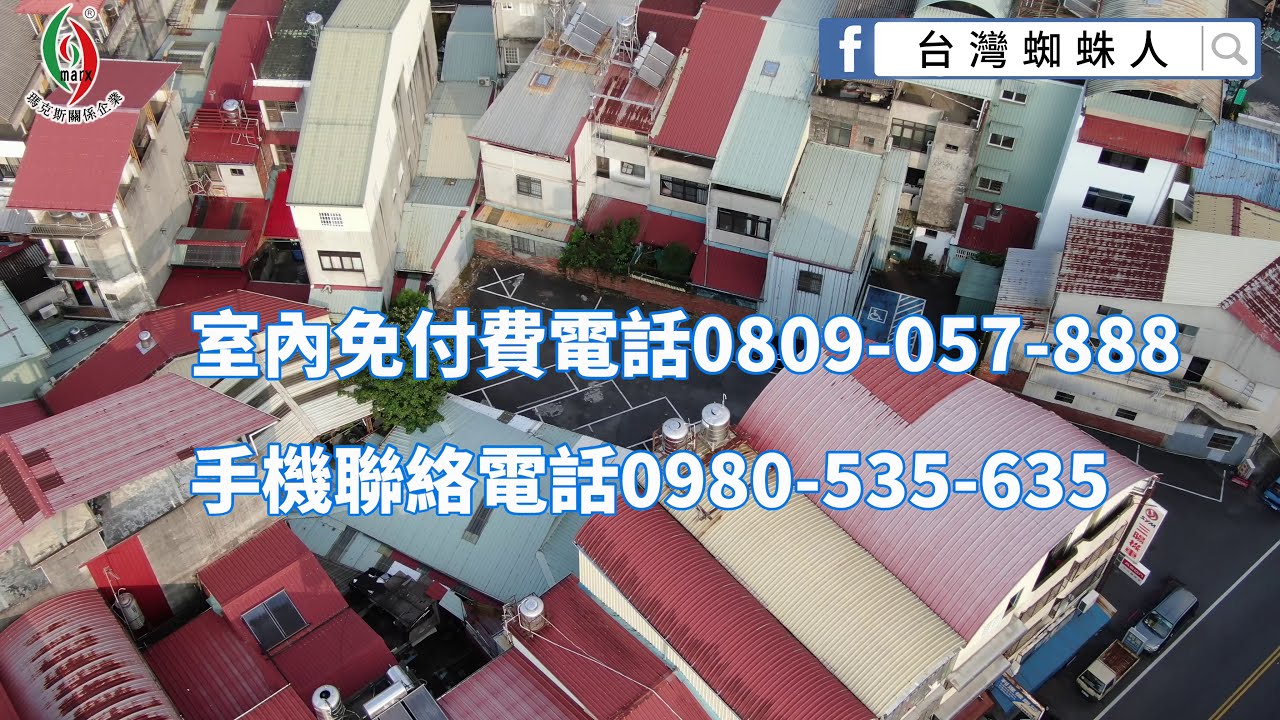This detailed aerial view, likely captured by a drone, reveals a densely packed residential area in an Asian country. The image showcases an intricate clustering of multi-story buildings, predominantly painted white with roofs ranging in colors from dark red and pink to beige and light gray. These roofs also feature varied designs including v-shaped, curved, and flat. The residential structures share walls but are offset, adding a patchwork aesthetic to the view. A small asphalt lot, which may serve as a parking area, is situated among the buildings, although no cars are evident there. However, several vehicles are visible near a street located in the lower right corner of the image. This street has two distinct yellow lines dividing it.

Superimposed on the photograph are lines of Chinese text. Centrally located is a prominent line containing the characters "0809-057-888", followed by another line with "0980-535-635". The upper right corner of the image features a strip with a recognizable Facebook logo adjacent to additional Chinese text and a search icon. The top left corner also contains a logo resembling two leaves with red and green swashes forming an oval shape, accompanied by more Chinese text. This visually rich photograph merges representational realism and typography, providing a comprehensive glimpse into the urban landscape and its informational overlay.